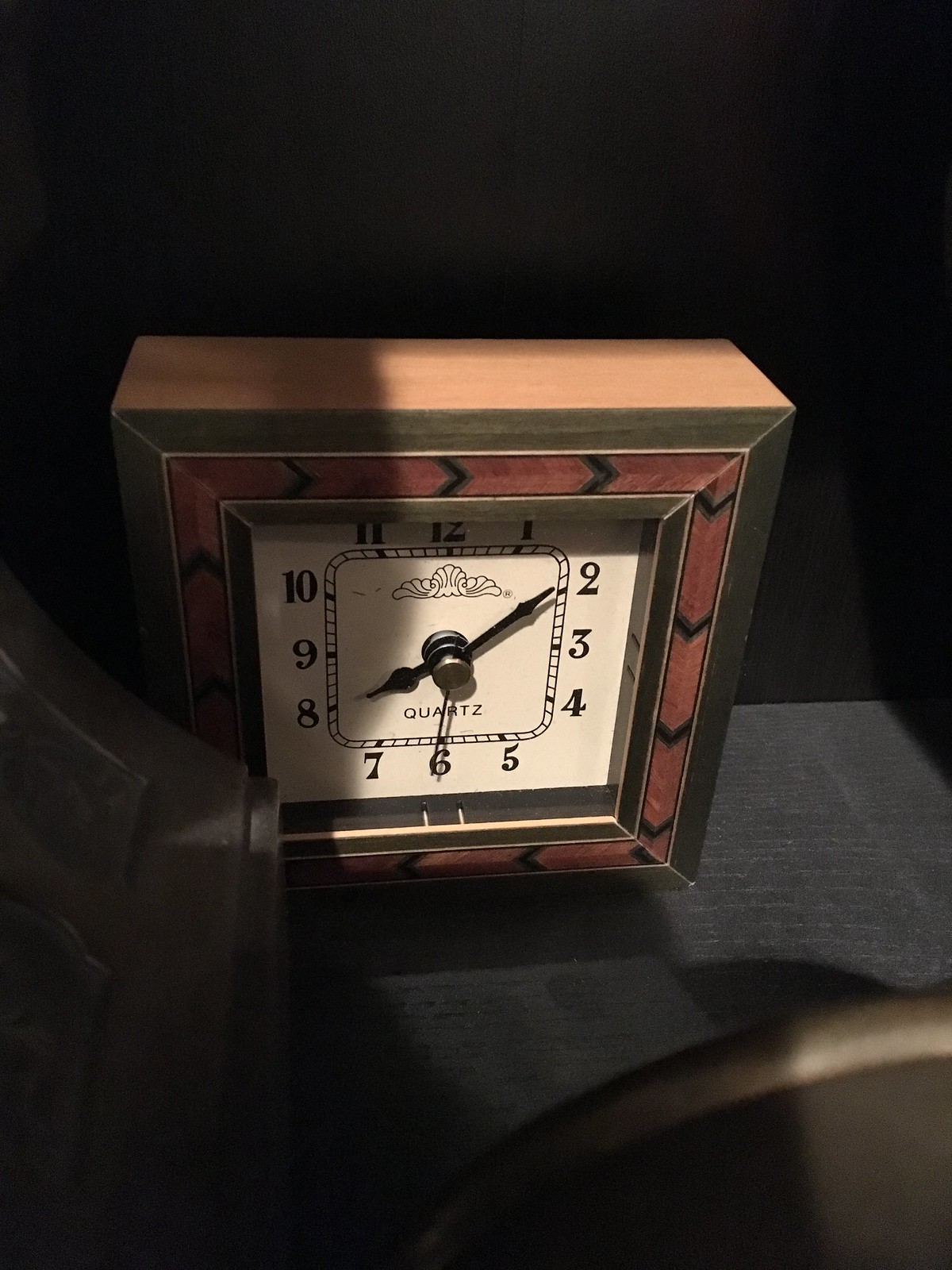This color photograph captures a square wooden clock sitting on a black cloth-covered table in the dark. The black cloth has a textured weave. The clock features different shades of brown wood: a light brown wooden exterior, a golden or dark brown painted frame, and a reddish-brown inner frame with black chevron designs. Shadows are cast on the clock from the top. The clock face is cream-colored with black numbers 1 through 12 arranged in a square pattern around the face. The black minute, hour, and second hands point to 8:10 and 30 seconds. Below the hands, the word "quartz" is displayed, and above them, there is a small black design resembling shells. A shadow falls at the bottom right of the image, adding depth to the scene.